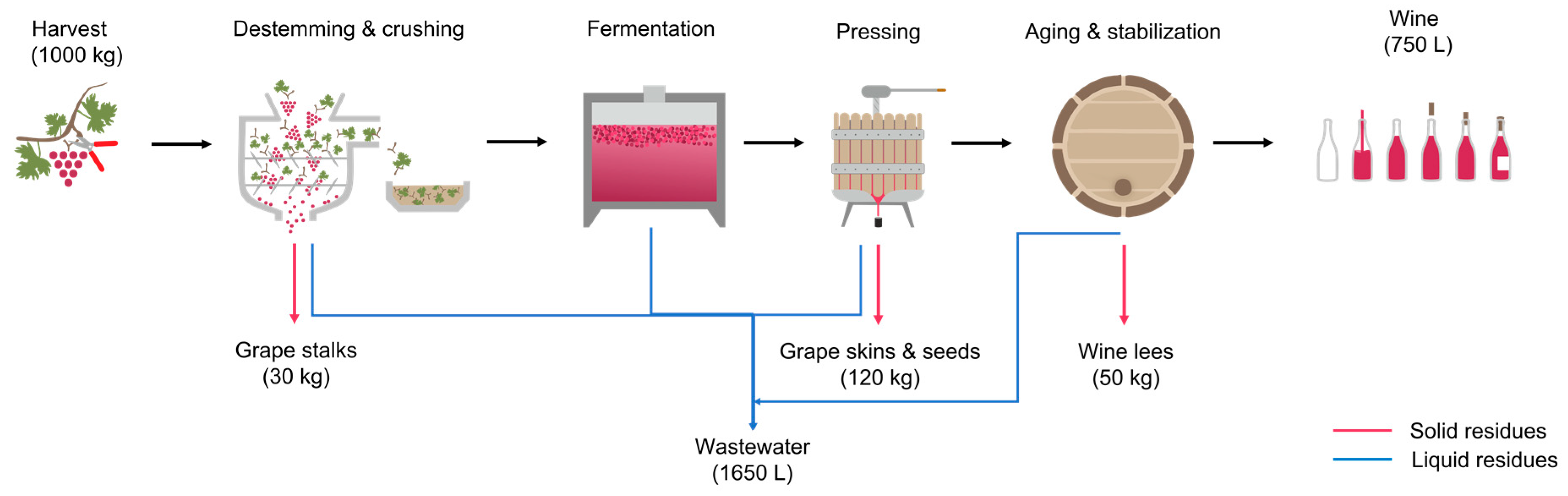The technical diagram illustrates the comprehensive wine-making process, starting from the harvest to the final bottling, using a sequence of connected clip art images and descriptive text. Starting on the far left, the diagram begins with the Harvest stage, depicting a grapevine and indicating a yield of 1000 kilograms of grapes. This leads to the De-stemming and Crushing phase, showing a machine processing the grapes and highlighting the byproduct of grape stalks with a pink arrow. Following this is the Fermentation stage, illustrated by a vat containing pink fermenting grape juice, with 1650 liters of wastewater noted as a byproduct. The next stage is Pressing, represented by a press machine, producing 120 kilograms of grape skins and seeds. The subsequent Aging and Stabilization stage is depicted with a wine cask, generating 50 kilograms of wine lees, shown via another pink arrow. Finally, the Wine stage features bottles with varying levels of wine, quantifying the output as 750 liters. Beneath the main production process, additional arrows indicate the byproducts: grape stalks, grape skins and seeds, wastewater, solid residue, and liquid residue, categorized with pink (solid residues) and blue (liquid residues) arrows. The entire process is visually tied together with arrows and lines, effectively mapping the journey from grape harvesting to the final production of wine.